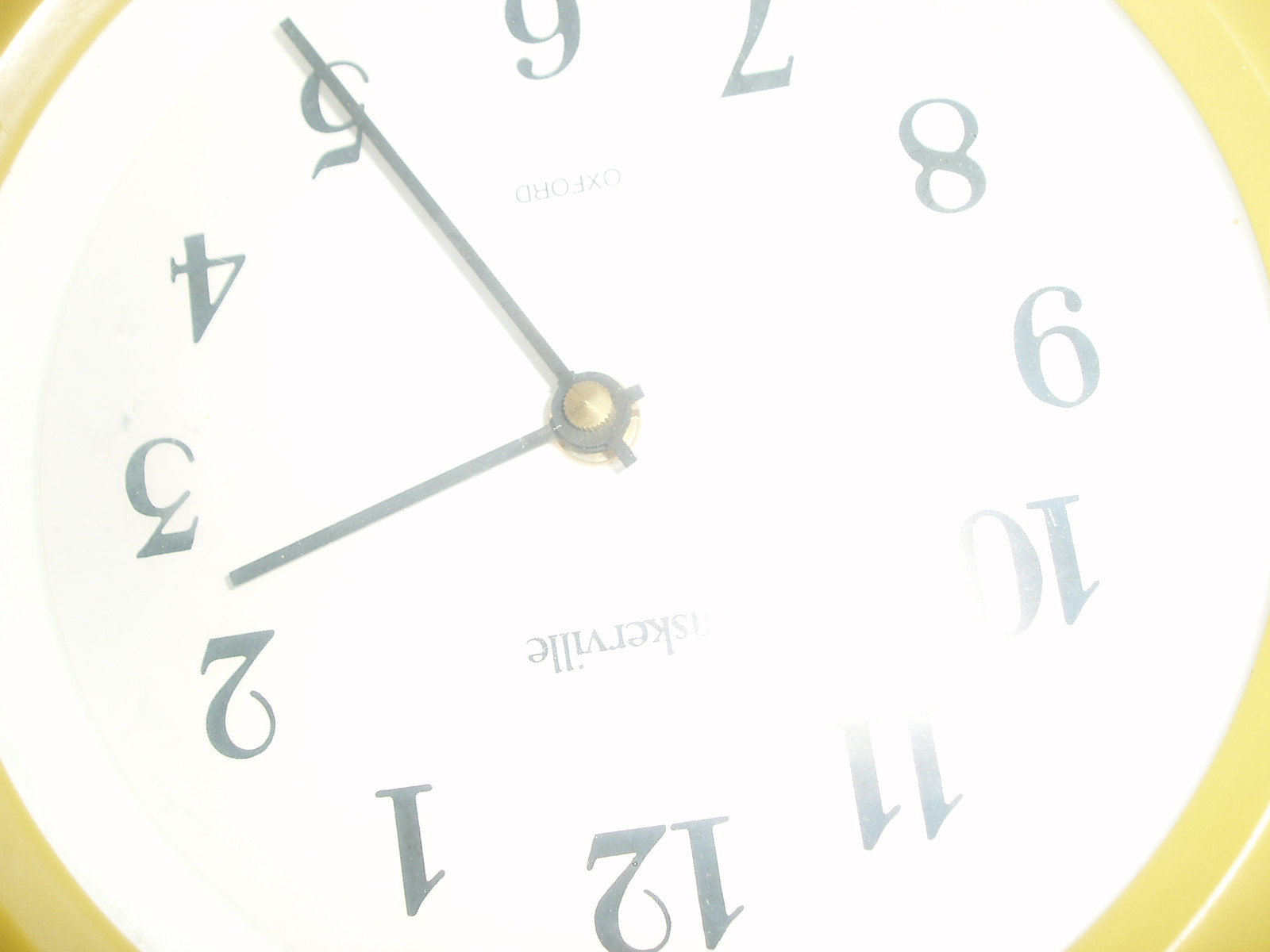This image features a vintage clock with a predominantly white face that appears slightly washed out. The clock is framed by a rounded yellow border, which is accented with a thin white detail line running along its inner edge. Notably, the clock is inverted, rendering all the numbers and inscriptions upside down. The numerals are black and clearly visible. Although the entire word at the top of the clock face is not fully legible due to the angle, the letters "S-K-E-R-V-I-L-L-E" can be discerned. Positioned beneath the brass fastener that holds the clock hands, the word "Oxford" is also visible in black.